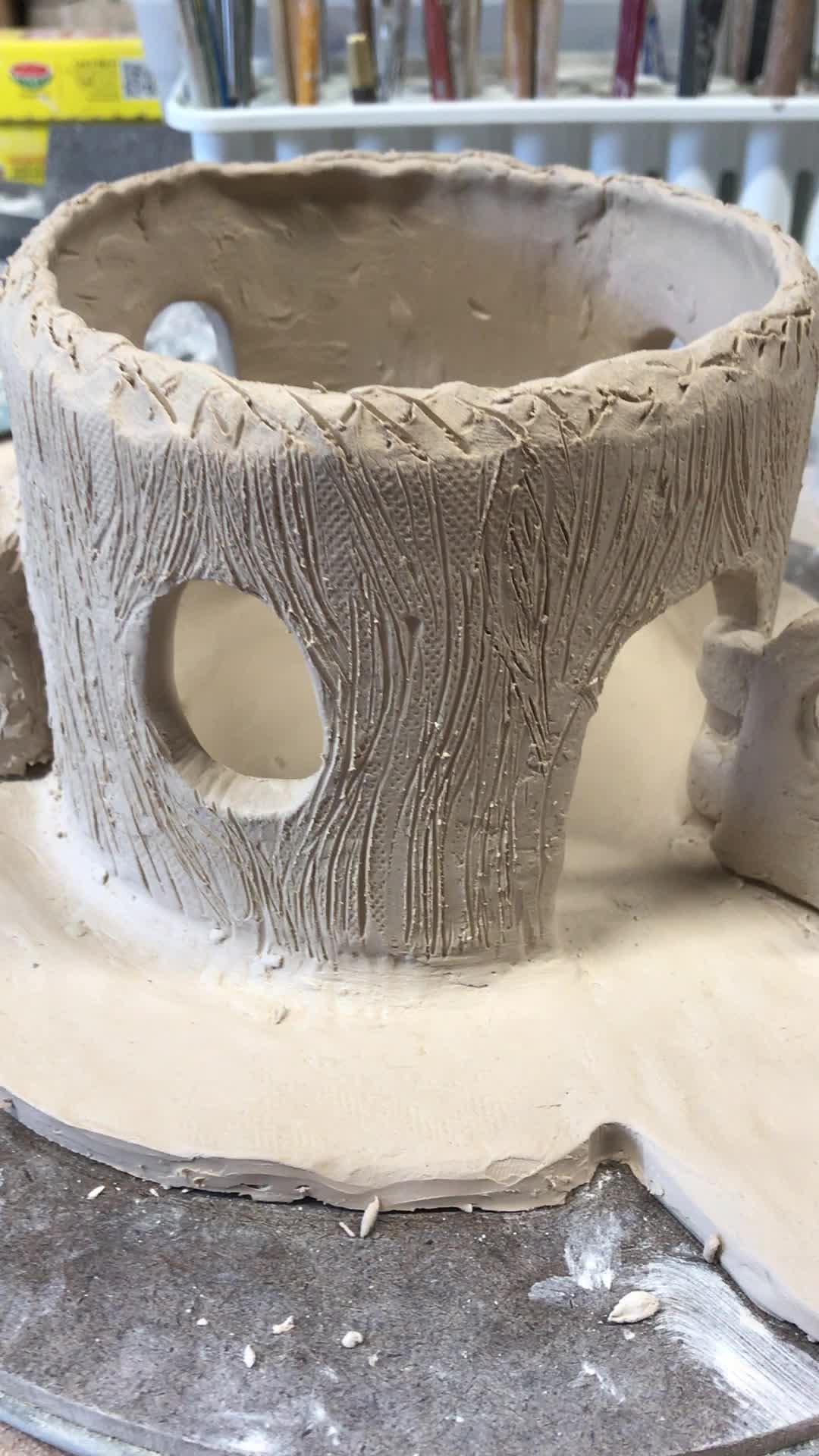The image captures a studio or workshop setting dedicated to pottery and clay sculpting. Dominating the background is an organized tool holder brimming with an assortment of tools, meticulously arranged in individual slots. Positioned centrally is an unfinished clay sculpture, resembling a circular house or tree trunk. This structure is distinctly roofless, revealing its hollow interior. The sculpture features meticulously crafted details such as circular window cutouts on the left and arched doorways on the right. Engraved lines adorn its exterior, mimicking the texture of logs, suggesting a tree house aesthetic. The sculpture is crafted from a gray, unfired clay material and rests securely on a potter's wheel, its white base accentuating its earthy tones.